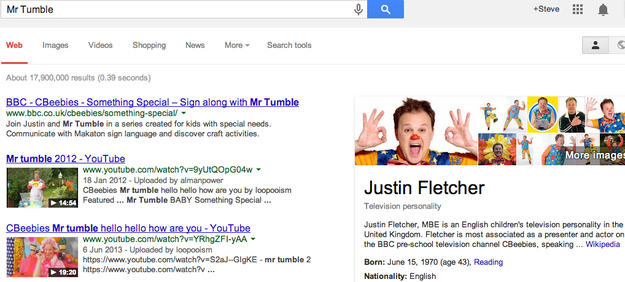The image showcases a Google search result on a white background, featuring various elements and links related to "Mr. Tumble." At the top, the search bar displays the term "Mr. Tumble," with icons for a microphone, a magnifying glass, a Google+ option labeled Steve, a menu icon, and a notification bell to its right. Below the search bar, the standard Google menu appears, offering options for Web, Images, Videos, Shopping, News, More (with a dropdown arrow), and Search Tools, followed by a user icon on the far right.

The search results indicate approximately 17,800,000 results, retrieved in 0.39 seconds. The first search result is a link to BBC's CBeebies show "Something Special," featuring a sing-along with Mr. Tumble. Brief information about the show accompanies the link.

The second result is a YouTube link to a video titled "Mr. Tumble 2012," displaying a thumbnail of a person standing in a grassy area, dressed in a vibrant, colorful outfit. The video has a runtime of 14 minutes.

The third result is another YouTube link titled "CBeebies: Mr. Tumble - Hello, Hello, How Are You?" The thumbnail shows a man with long blonde hair in a playroom with colorful decorations, clad in pink. The video is 18 minutes long.

On the right side of the image, there is a sidebar featuring information about Justin Fletcher, the actor who portrays Mr. Tumble. His main picture shows him with an enthusiastic expression, making an "OK" sign with both hands while wearing a red clown nose. He is identified as a Caucasian male with brown hair, aged 43. A collage of additional pictures of Justin Fletcher is present beneath the main image. The sidebar text elaborates on his background, stating that he is an English children's television personality from the UK, born on June 15, 1970, with a nationality of English.